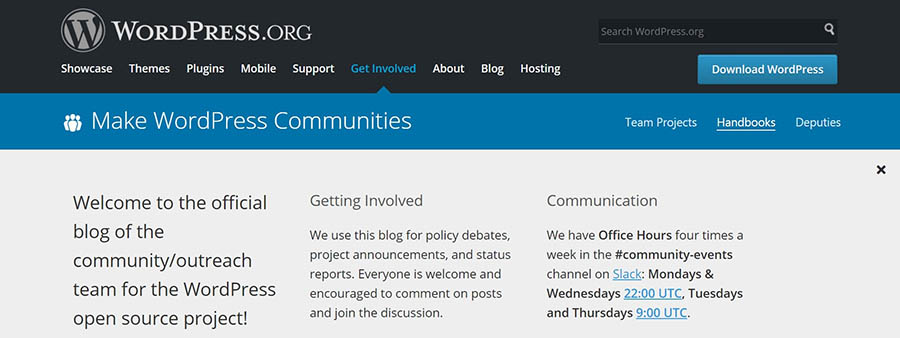**Homepage of WordPress.org**

This is a detailed screenshot of the homepage for WordPress.org, the world's most renowned blogging platform, especially prominent in English-speaking regions, though likely supporting a variety of languages. 

The page features a sleek, dark gray header that includes the following menu options: Showcase, Themes, Plugins, Mobile, Support, Get Involved, About, Blog, and Hosting. The "Get Involved" option is highlighted with a blue triangle beneath it, indicating it as the current selection, with the text itself also in blue. On the right side of this header, there is a search bar labeled "Search wordpress.org."

Just below the header, there is a prominent blue button labeled "Download WordPress" for users seeking to install the platform.

In the "Get Involved" section, which we delve deeper into, there is an icon featuring three figures resembling bowling pins, symbolizing community engagement. This section highlights several key areas:
- **Make WordPress Communities**
- **Team Projects**
- **Handbooks** (with "Handbooks" being emphasized by an underline)
- **Deputies**

Below this, the content is organized into three columns. 

The left column features a welcoming message in large text: "Welcome to the official blog of the Community Outreach Team for the WordPress Open Source Project!"

The middle column, "Getting Involved," explains the blog's purpose:
- It is used for policy debates, project announcements, and status reports.
- Everyone is encouraged to participate by commenting on posts and taking part in discussions.

The right column, "Communication," details the community's office hours, held four times a week in the #Community-Events channel on Slack:
- Mondays and Wednesdays at 2200 UTC
- Tuesdays and Thursdays at 0900 UTC

This comprehensive overview provides a clear and inviting glimpse into the WordPress.org homepage and its community engagement features.